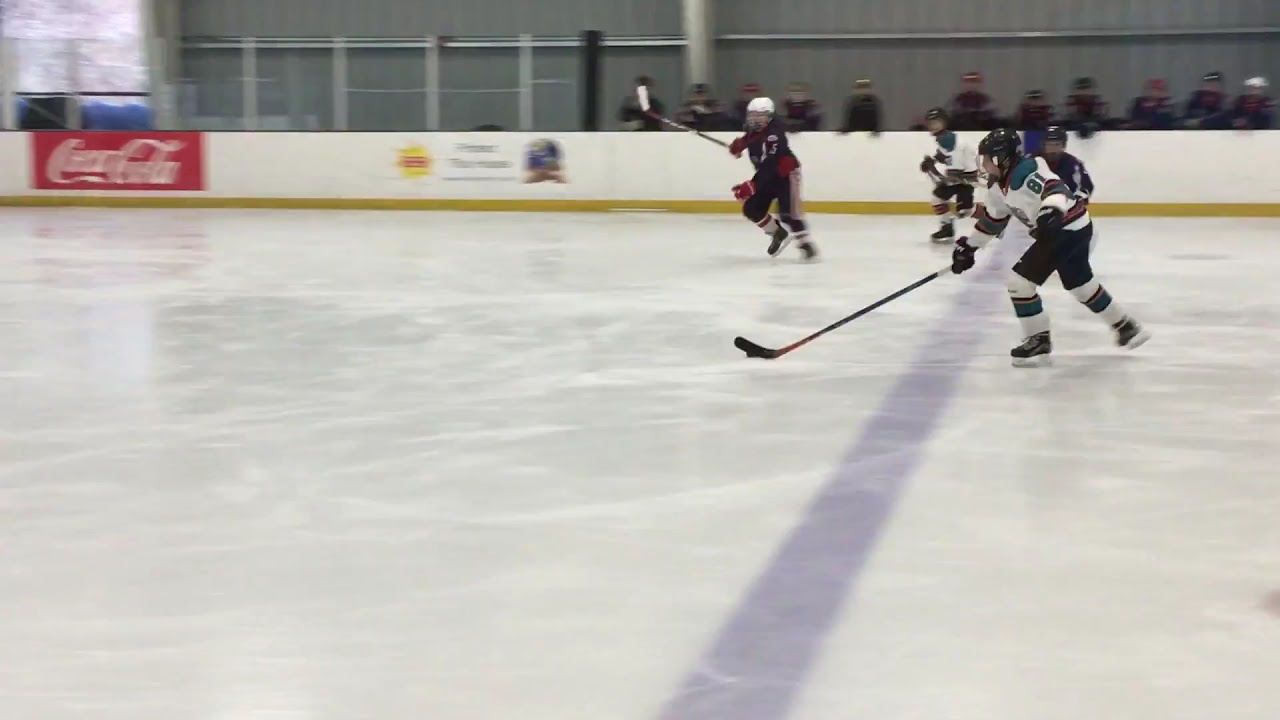In the center of the ice rink during a dynamic hockey game, the close-up shot captures players in motion. The rink is framed by a blurry background of spectators and a prominent Coca-Cola sign in white against a red backdrop on the right wall. The ice, pristine and white, features a distinct purple line running across its surface. In the foreground, a hockey player in a white jersey adorned with green accents and the number A1 on the back faces the camera, poised with his stick next to a visible puck. His team’s uniforms contrast with opposing players farther back, seen in red and black attire. To his left, another player in a black helmet and white jersey with the number 81 prominently displayed on the shoulder also wields a hockey stick, ready for action. The players are surrounded by a fence lined with various signs, and beyond that, a blurry throng of spectators eagerly watches the intense game unfold.